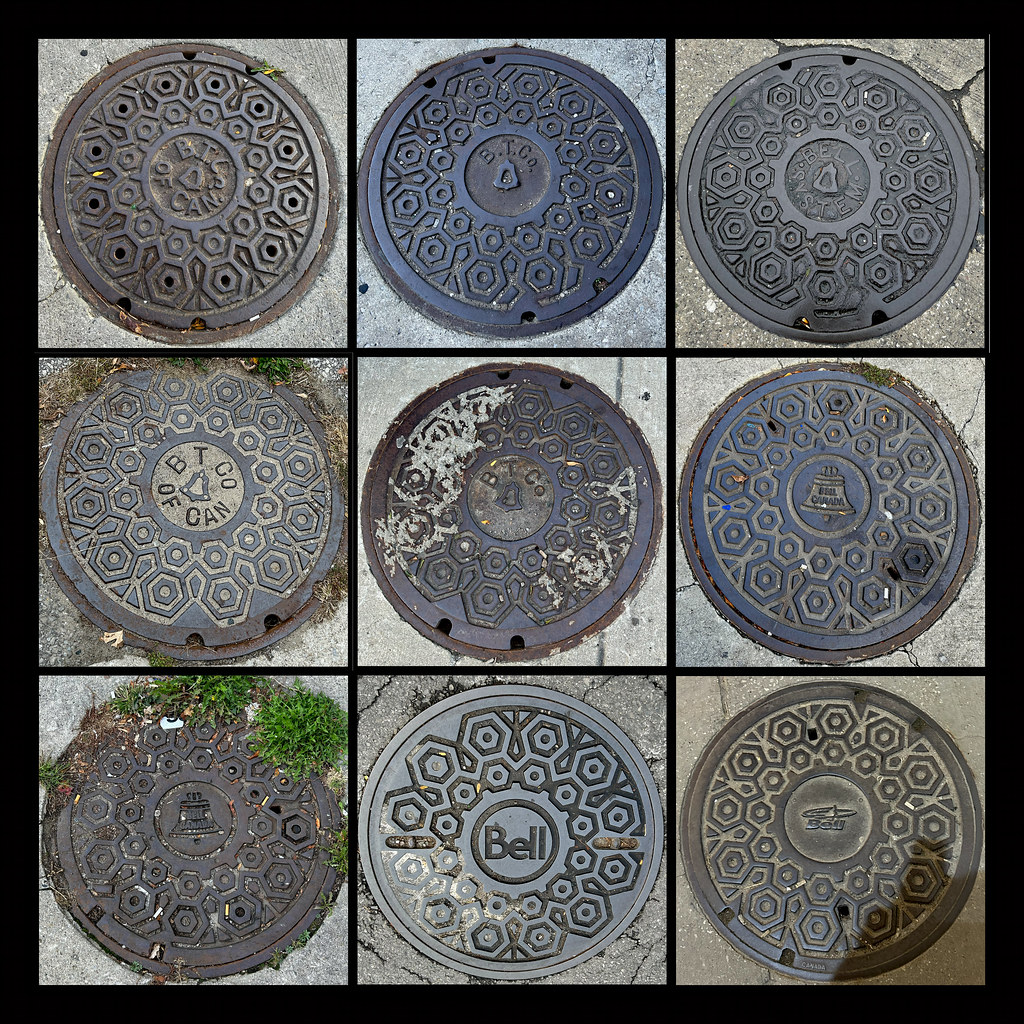This is a detailed colour photograph presented as a composite illustration of nine different manhole covers arranged in a three-by-three grid. Each manhole cover is round and depicted in its unique state, forming a visually engaging montage. The image is bordered by a thick black rim, and each individual photograph within the square grid is separated by thinner black lines.

The manhole covers show a range of conditions and details. Notably, the cover in the bottom left corner is surrounded by green weeds and grass, making it more difficult to discern the pattern on its dark, dirty metal surface. The bottom middle cover stands out for its cleanliness, prominently displaying the word "Bell" etched into its metal surface. Another cover, located in the middle left, has writing around the circumference of an inner circle, with the letters "BT," "CO," "OF CAN," and a bell icon engraved in the center, revealing its association with the Bell Telephone Company of Canada.

Some covers exhibit signs of wear and possibly neglect, with a few appearing slightly caved in. For instance, the cover in the middle is not completely flat, as it is sunken on the top left corner. Other covers show various shades of grey, ranging from light to bluish-grey, with different embossed designs. The pavement surrounding the manholes also varies, with some areas showing cracks and signs of wear. The bottom right cover includes a shadow in the bottom right-hand corner, adding to the depth and texture of the overall image. The composite not only captures the utilitarian nature of these street features but also highlights their diverse states and subtle details.